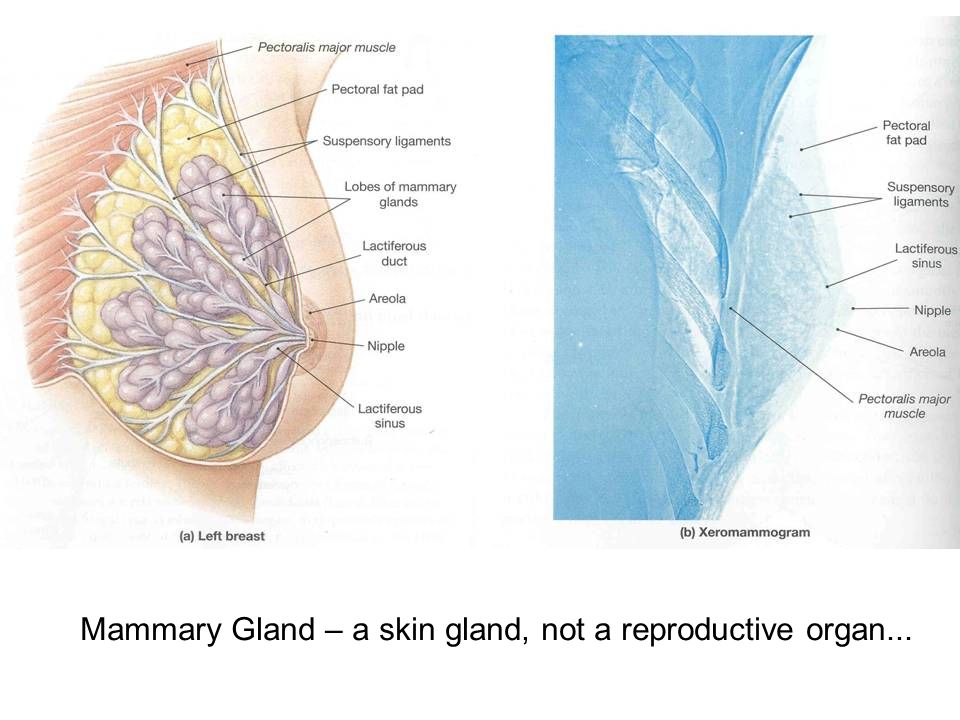The image is a detailed anatomical illustration of the mammary glands with both a scientific drawing and a mammogram on a white background. The left side features a labeled side-view cutaway of the left breast, highlighting the pectoralis major muscle, pectoral fat pad, suspensory ligaments, lobes of mammary glands, lactiferous duct, areola, nipple, and lactiferous sinus. At the bottom, it is labeled "Left Breast" and in the top right corner, it says "A". On the right side, labeled as "B" and "Zero Mammogram" beneath, there is a mammogram image of the breast showing the same structures such as the pectoral fat pad, suspensory ligaments, lactiferous sinus, nipple, areola, and pectoralis major muscle. At the bottom of the image, it states in black letters: "Mammary gland - a skin gland, not a reproductive organ."